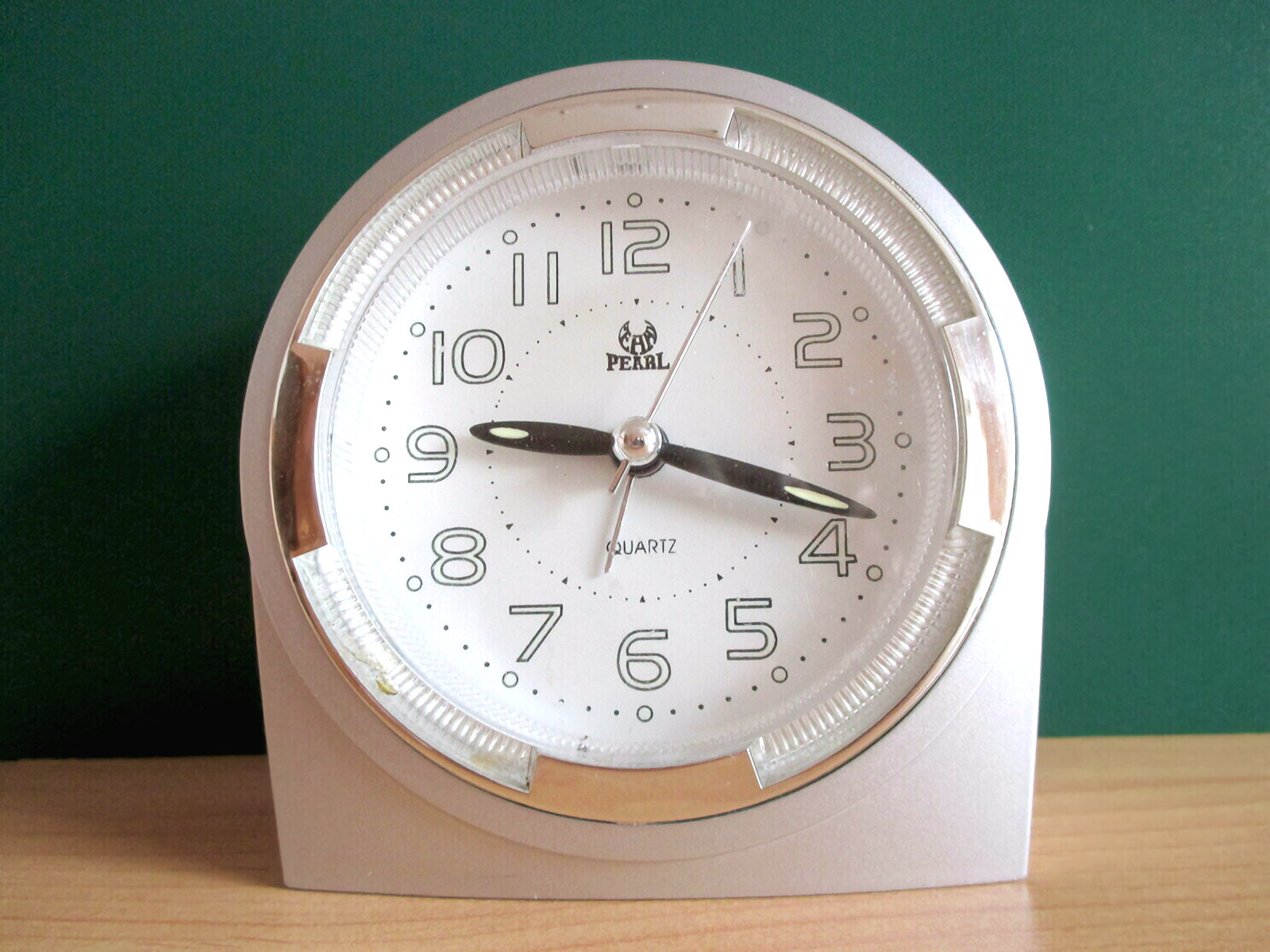A small, white clock is sitting on a woodgrain table, likely made of formica. The clock features a rectangular base that smoothly transitions into a curved top, harmonizing with the round shape of the clock face. The clock face itself is white, displaying numbers 1 to 12 outlined in black. Each number is filled with white within its black outline. Around the edge of the dial, there are small circles marking every five-minute interval and dots or dashes for each one-minute increment. The time-telling is facilitated by oval-shaped black hands for hours and minutes, each tipped with a glow-in-the-dark patch. A slender silver second hand completes the time-keeping trio, accurately indicating that the current time is 9:18 and 5 seconds. Behind the clock stands a rich, dark green wall, providing a stark and elegant contrast to the scene.